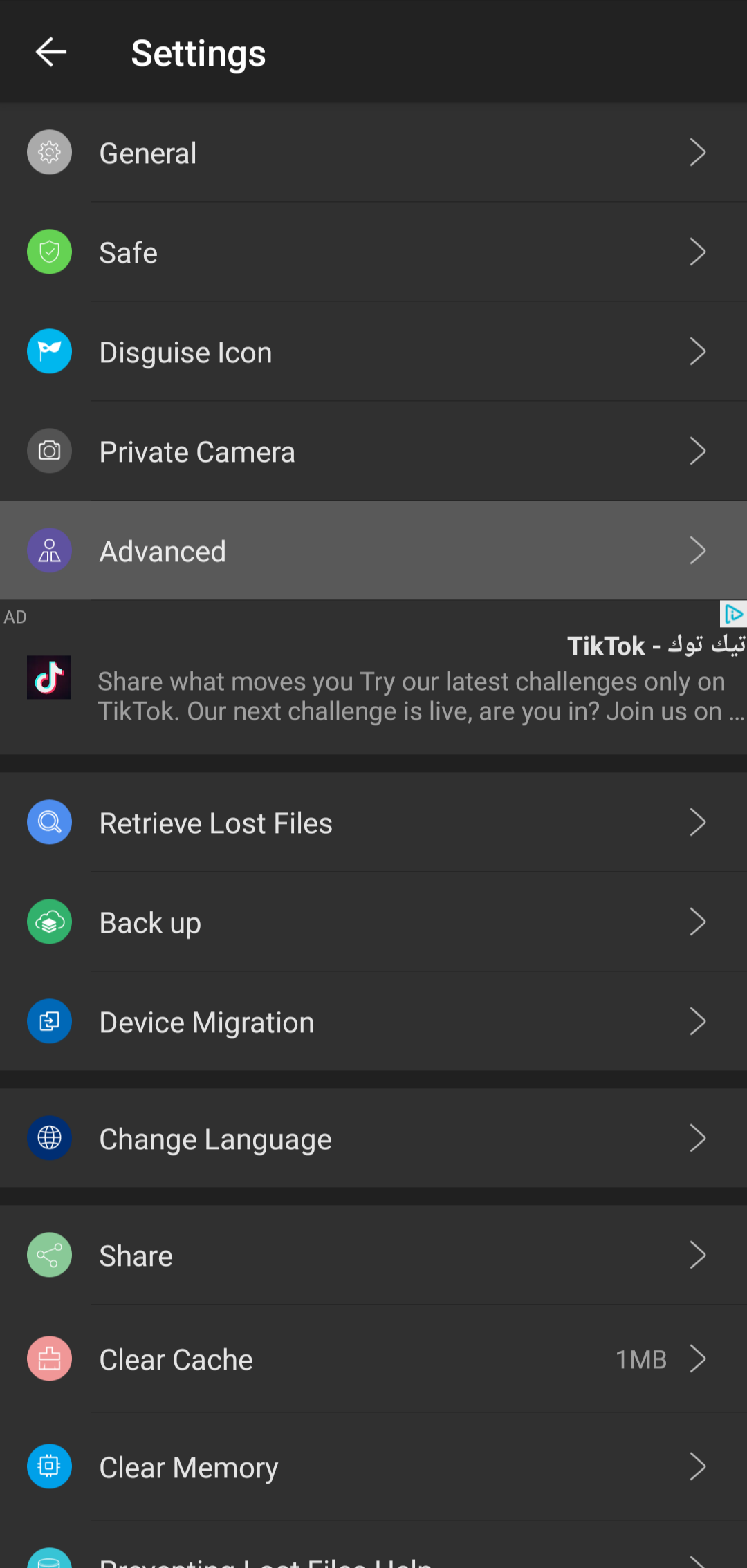The image is a screenshot of the settings page on a smartphone displaying in dark mode, characterized by a very dark gray, nearly black background. At the top left of the screen, the word "Settings" is written in a white font, accompanied by a white left-pointing arrow. Below this header, there is a vertical list of settings options, each accompanied by a small, oval-shaped icon. The visible settings in this section include:
1. General
2. Safe
3. Disguise Icon
4. Private
5. Camera

A gray-bordered section titled "Advanced" then interrupts the list. Below this delineated section, the typical settings background resumes, and an advertisement featuring the TikTok logo appears. The ad text reads: "Share what moves you, try our latest challenges only on TikTok. Our next challenge is live, are you in? Join us on..." However, the remainder of the message is obscured and not visible in the screenshot. 

Following the ad, the settings list continues with additional options:
1. Retrieve Lost Files
2. Backup
3. Device Migration
4. Change Language
5. Share
6. Clear Cache
7. Clear Memory

The inclusion of an advertisement within the settings menu is noteworthy, adding an unexpected element to the page layout. The screenshot does not display the phone's top border, thus omitting the time and battery status indicators.